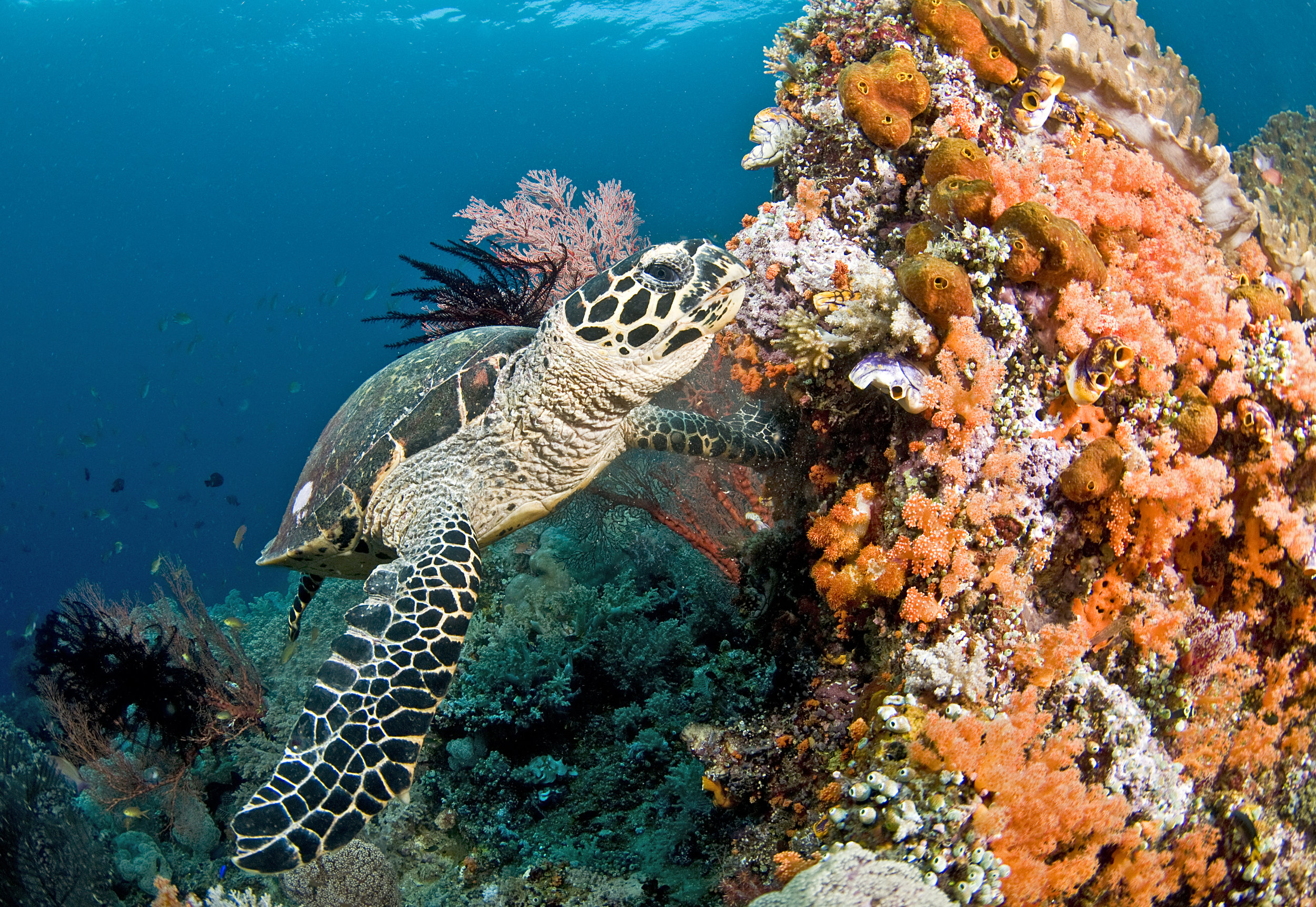In this photographic underwater image set in the ocean, a sea turtle is swimming gracefully from the bottom left to the top right. The turtle, centered on the left side of the frame, has a distinct white head speckled with black spots and a sharp beak. Its dark shell, appearing almost black or very dark green, contrasts with its front flippers, which are marked by intricate white, web-like patterns over a black background. The turtle's flippers are spread open as it moves through the water. 

To the right of the turtle, occupying almost half of the image from the bottom right-hand corner to the top right-hand corner, is a large coral reef. This coral reef is a vibrant mix of colors and textures, featuring hues of orange, white, gray, greenish-blue, and some additional purple, red, pink, and reddish formations that give it a rugged, rocky appearance. Various coral types, including softer growths and barnacles, cover the reef, adding to the complexity of the scene.

In the bottom left-hand corner, a small fish swims near some black underwater plant material. The image background transitions from the deep blue of the ocean in the lower parts to a lighter blue near the surface at the top left, indicating the progression towards the ocean surface. There is no text within the image, allowing the natural beauty of this underwater scene to take center stage.